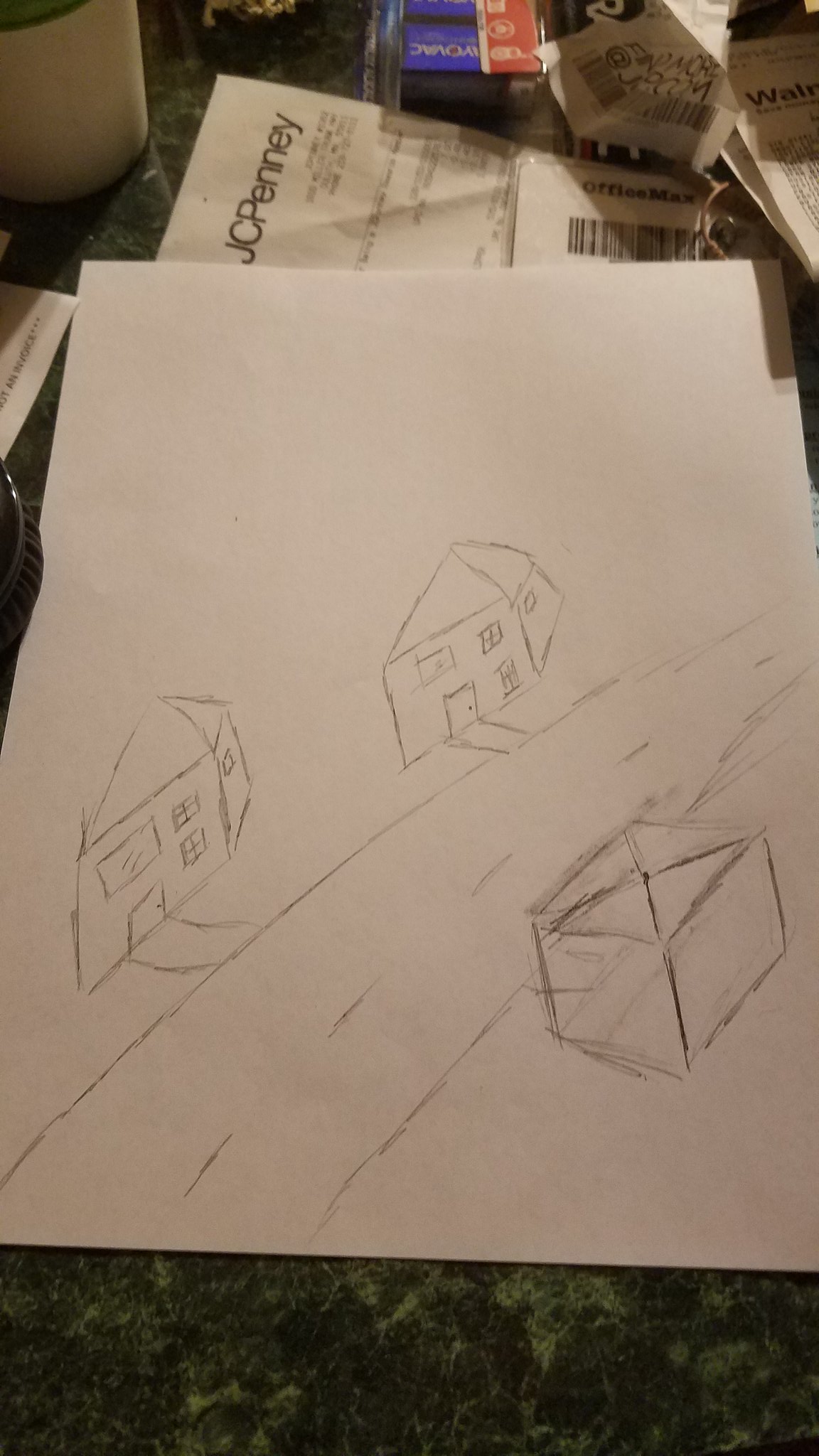A detailed view of a gray desk or checkout counter is depicted in this image. In the background, a row of small boxes is visible, each sporting blue on one end and red on the other. Prominently displayed on the desk is a large, round container. To the side, a small white piece of paper is noticeable. Lying near it is a JCPenney receipt, white with black print, alongside a product barcode, also rendered in black print on white. Additionally, a large piece of paper is spread out on the desk, featuring a drawing in black pencil. The sketch includes a box, a couple of houses, and a road, meticulously detailed in monochromatic hues.